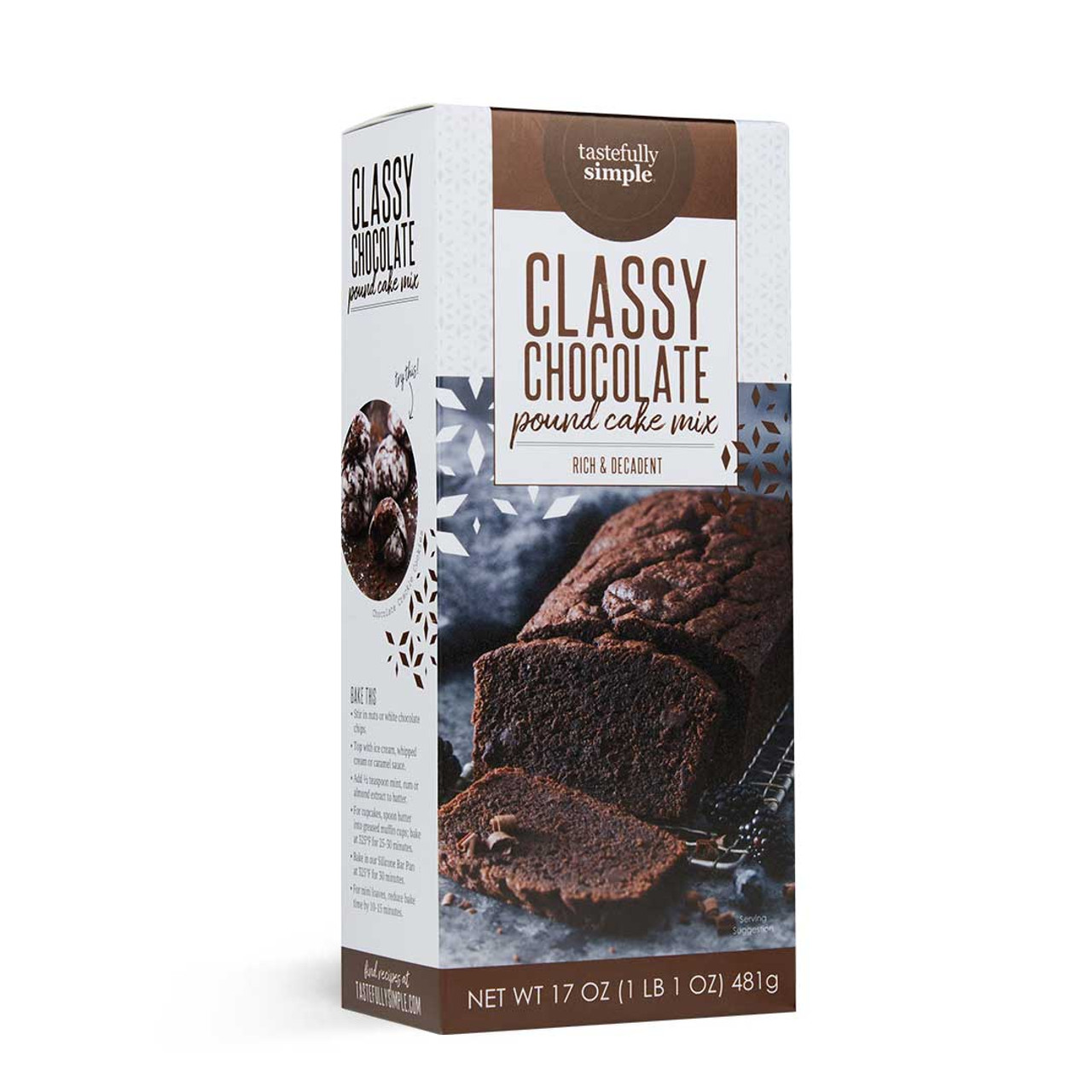The image features product packaging for a "Classy Chocolate Pound Cake Mix" by Tastefully Simple. The box, which resembles the shape of a milk carton but with a flat top, stands against a pale blue and gray background with a vintage aesthetic. At the top of the packaging is a black-brown text box with the text "Tastefully Simple" in white. Below this, in brown lettering, the product name "Classy Chocolate" and "Pound Cake Mix" is prominently displayed. The packaging boasts that the product is "rich and decadent." An inviting image of a chocolate pound cake, with two slices cut from it, is featured on the front. The cake sits on a metal rack surrounded by blueberries or blackberries. The left side of the box mirrors the front with repeated text and additional features such as another product that can be made with the mix and some directions for preparation. The design is completed with a brown trim near the bottom of the packaging. Additionally, the weight of the cake mix is displayed on the left side of the box.